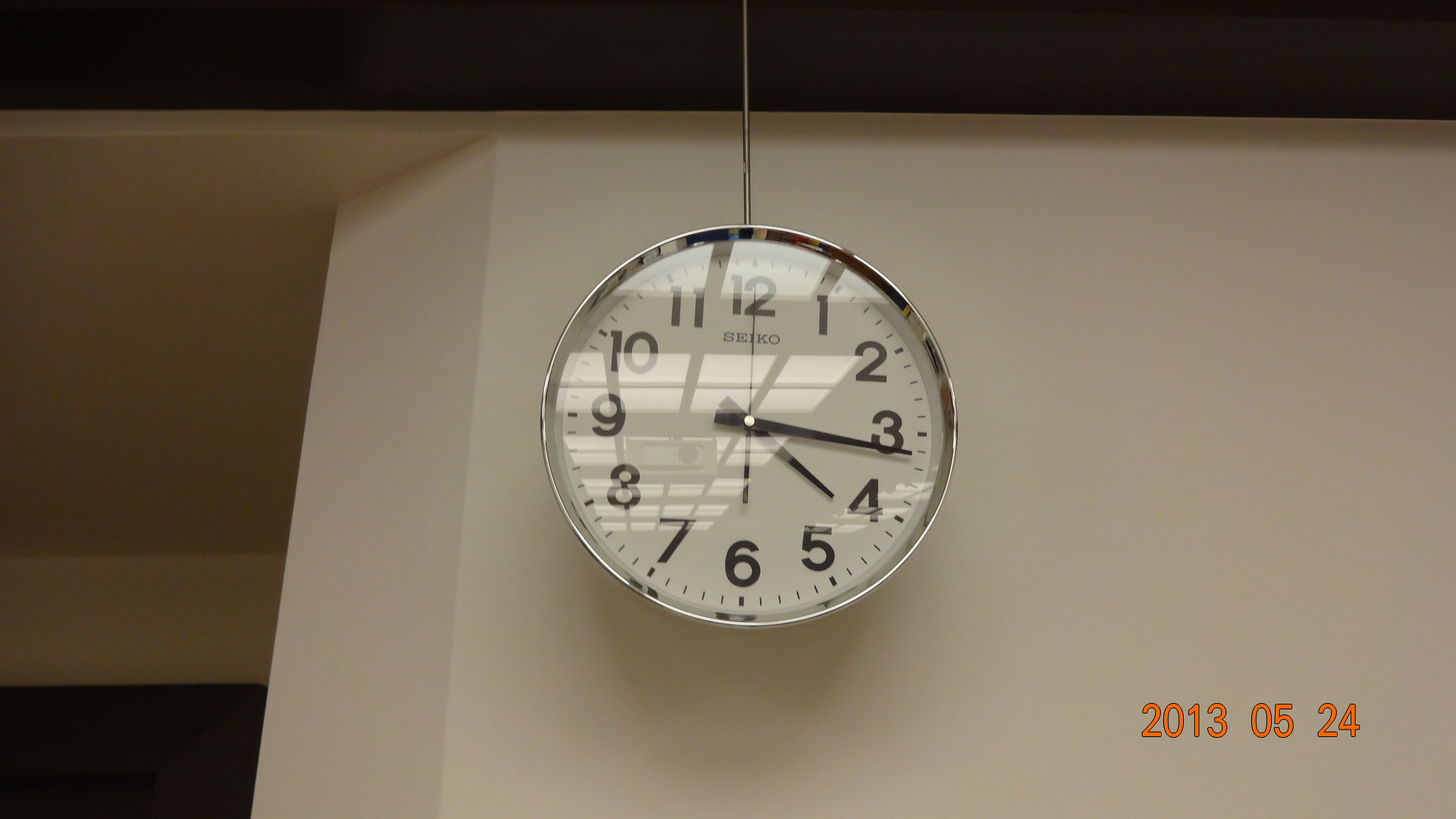This image features a round wall clock with a silver frame, hanging from the ceiling on a thin metal rod. The clock is situated against a white wall, with an open doorway visible on the right side, leading into another room. The setting appears to be an office rather than a house, as evidenced by the reflection of numerous overhead neon lights, typically found in office cubicles, on the clock face.

The clock itself has a white face with black numerals arranged in the standard sequence from 12 to 11. The time displayed is approximately 4:16, with the black hour and minute hands positioned accordingly and the second hand pointing at the 6 o'clock mark. Notably, the image contains a date stamp in the bottom left corner, indicating "2013 5-24," which corresponds to May 24, 2013. This detail, combined with the glare from the overhead lights and the clock's reflections, adds a layer of complexity to the otherwise straightforward depiction of a timepiece.